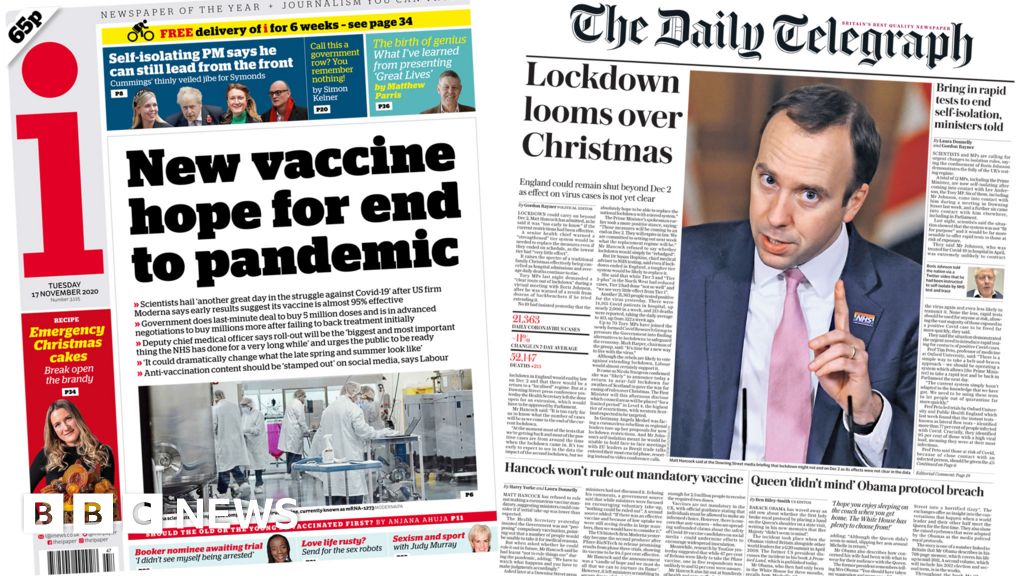The image depicts a copy of the Daily Telegraph newspaper. The front page prominently displays a headline about the Prime Minister, who, despite self-isolation, asserts his capability to lead effectively. 

In the top left corner, the newspaper is noted as costing 65p and is labeled "Newspaper of the Year." A promotional offer for free delivery for six weeks can be seen on page 34. 

A large red "I" indicates a significant story about a new vaccine, sparking hope for an end to the pandemic. Another headline mentions the availability of "emergency Christmas cakes."

There are white squares with black lettering that spell "BBC," situated above a barcode. The adjacent page carries more headlines and articles, stating, "The Daily Telegraph: lockdown looms over Christmas," suggesting that England might remain under restrictions beyond December 2nd and possibly into the new year. One article calls for rapid testing to end self-isolation, quoting “my meter's told.”

Additional headlines at the bottom reveal that Health Secretary Hancock has not dismissed the idea of mandatory vaccinations, and there is a mention of the Queen's unperturbed reaction to former President Obama's protocol breach.